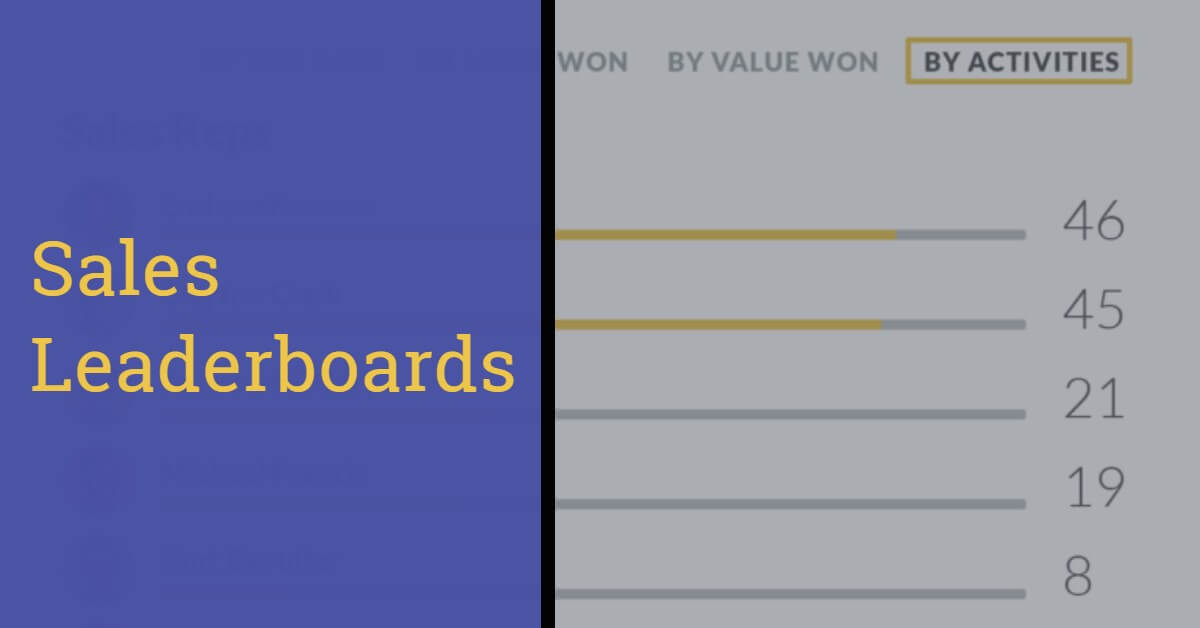In the image, the left side features a medium blue box with the title "Sales Leaderboard" in yellow letters, reminiscent of the Jeopardy blue color. The right side of the image resembles a white computer screen or a postcard-like card. At the top of this section, it is labeled "By Activities." Beneath this title is a series of progress bars representing the sales activities rankings. The top two entries show significant progress, with the first place at 46 and the second at 45, both nearly fully highlighted in yellow. The subsequent rankings are 21, 19, and 8, with their respective progress bars entirely empty, indicating no visible progress. The overall layout appears to be part of a presentation slide in muted colors, contrasting with the blue and yellow elements on the left.